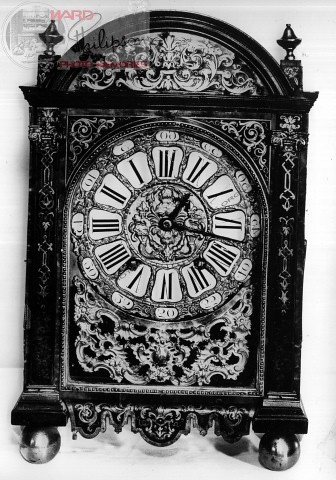The black and white image showcases an old-fashioned clock, rendered in shades of black, white, and gray. The clock's body stands vertically, supported by round ball feet at the base. The top of the clock features a gracefully curved arch adorned with intricate, ornate designs that extend down its sides, creating an elegant appearance. Nestled within an inset curved arch, the clock face stands out with its peculiar Roman numerals. The numerals appear to repeat and are arranged in a nonsensical order. Despite the unusual sequence of numerals, the clock still possesses a functional hour hand and second hand. The craftsmanship and unique character of the clock are beautifully highlighted in this thoughtfully composed, monochromatic image.